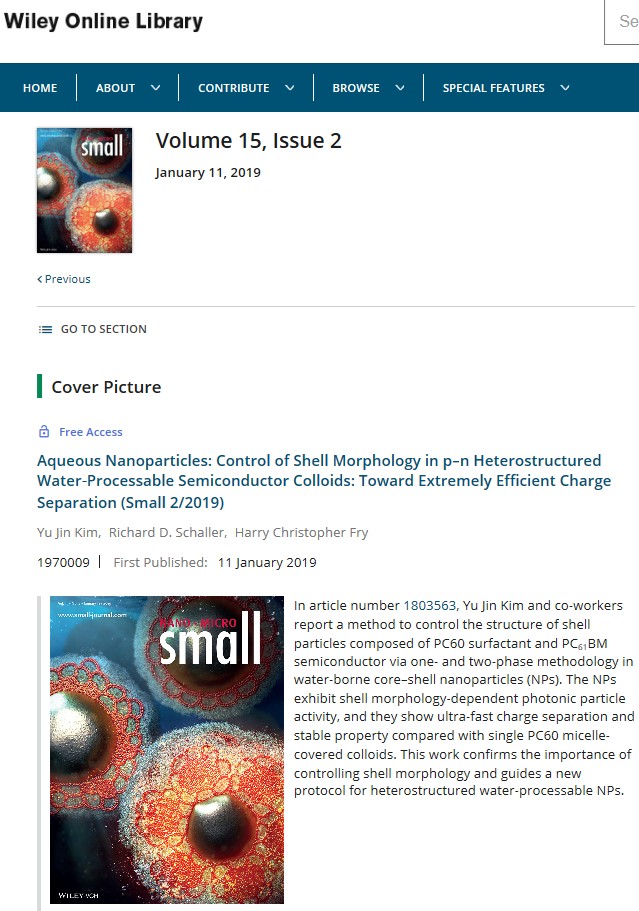**Descriptive Caption:**

On a white background, the top section of the image prominently displays the "Wiley Online Library" logo. In the upper right corner, there is a small box with "SE" inside. Below this, a dark blue navigation bar stretches across the width of the image, containing dropdown menus labeled "Home," "Contribute," "Browse," and "Special Features." 

Beneath the navigation bar, a smaller area shows "Volume 15 Issue 2 | January 11th, 2019," accompanied by a back arrow labeled "Previous." Below this, there are three bullet points titled "Go to Section," followed by a green line and the words "Cover Picture." 

An adjacent lock icon indicates "Free Access" to the featured article. The cover image description reads: "Aqueous nanoparticles control of shell morphology in P to N heterostructured water processable semiconductor colloids toward extremely efficient charge separation," attributed to "Small 2, 2019" along with the first publication date of "January 11th, 2019."

Further down, a long light blue line and the word "Small" are displayed again, alongside three circular icons with dark centers. The rest of the space is dedicated to details about the research and the authors involved in the work.